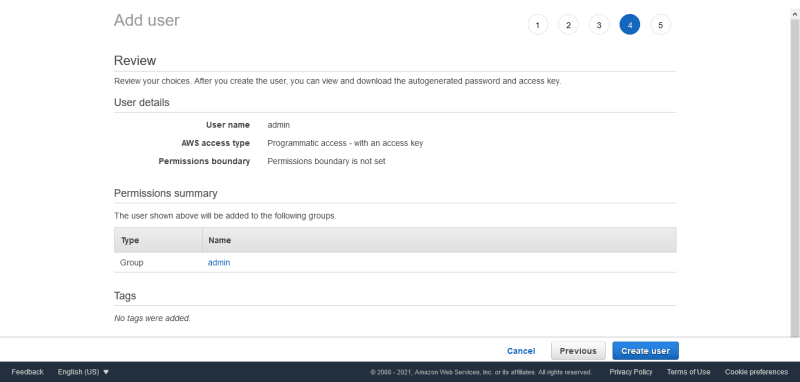Cropped Screenshot of User Addition Panel in an Ad Interface

The image is a cropped screenshot depicting an "Add User" panel within an advertisement interface. At the top left, in large, light gray letters, it reads "Add User." To the right, a horizontal line of numbered circles from 1 to 5 is displayed, with the number 4 highlighted, indicating that this is the fourth step in the process.

Beneath "Add User," the word "Review" is written in bold black letters, followed by the instructions "Review your choices. After you create the user, you can view and download the auto-generated password and access key."

Further down, under a section labeled "User Details," three fields are listed to the left: "Username," "AWS Access Type," and "Permissions Boundary." Correspondingly, to the right:
- The field beside "Username" shows "admin."
- The field beside "AWS Access Type" indicates "Programmatic access with an access key."
- The field beside "Permissions Boundary" states "Permissions boundary is not set."

Below the user details, there is a section titled "Permissions Summary" in dark gray letters. It mentions, "The user shown above will be added to the following groups," and lists a group type as "Group" and the group name as "admin."

Towards the bottom, under the "Tags" section on the left, it states "No tags were added."

At the bottom right of the screen, there are three clickable options: "Cancel," "Previous," and "Create user." "Create user" is highlighted in a blue box, "Previous" is in a gray box, and "Cancel" is emphasized in blue text.